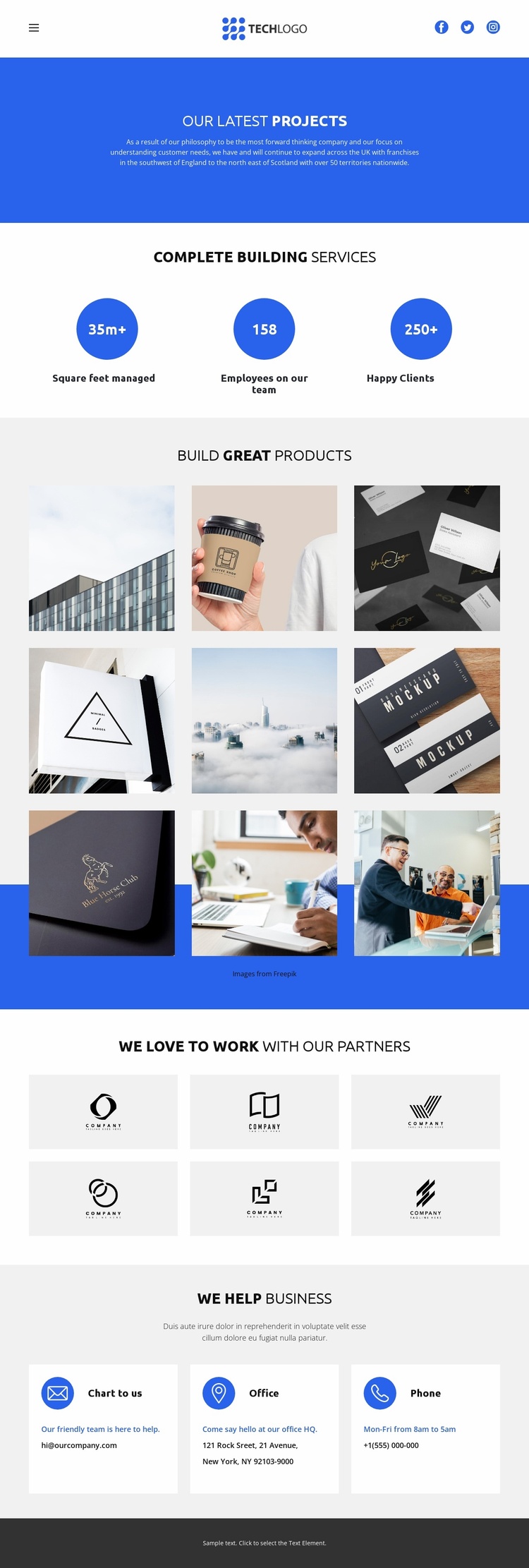A screenshot from what appears to be a travel website, displayed in portrait mode with a predominantly white background and accentuated by a cobalt blue theme, draws attention with its organized layout and vibrant design elements. At the top, a thick cobalt blue bar with the bold, white text "Our Latest Projects" captures immediate focus. Above this bar, a thin white margin features a blue logo accompanied by the text "Techie Logo," possibly indicating a graphic design or logo creation company. This margin also hosts three white-on-blue icons, with the top right icon identifiable as a Facebook symbol while the others remain unclear.

Directly below the cobalt blue bar is a white section labeled "Complete Building Services," presenting three selectable options. These options are highlighted by cobalt blue ovals with white text, one of which notably reads "35M+," while the others are not distinctly labeled.

The central portion of the screenshot showcases a structured collage consisting of three columns and three rows, totaling nine photographic images. These images range from a person holding a branded cup and business cards on a desk, to the rooftop of an industrial building and individuals shaking hands, suggesting a business-centric theme with a mix of real photos and clip art-like visuals.

Following the collage, the heading "We love to work with our partners" introduces two rows of partner logos, arranged in three columns per row, making up six logos in total. Each logo is positioned within a pale gray rectangle, although their details are not clearly readable.

At the bottom section, another descriptive area promotes business assistance, featuring three white boxes with blue circular icons, each accompanied by brief text descriptions that are not entirely legible. The page concludes with a solid black bar at the bottom, serving as a definitive end to the overall layout.